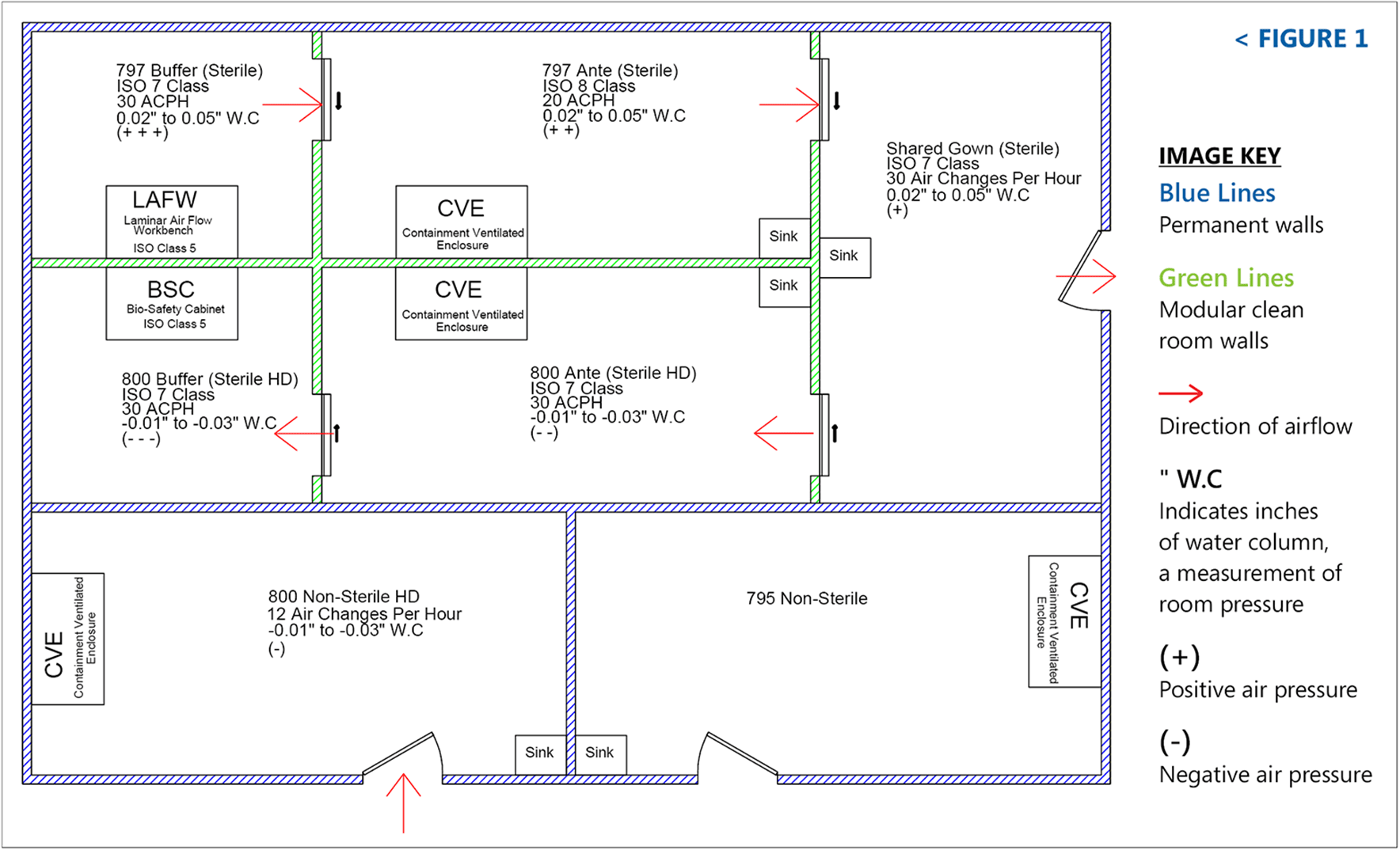The image is a detailed, white digital blueprint of a building design, outlined by a very thin gray border. The blueprint features a total of seven rooms – five smaller rooms positioned at the top and two larger rooms at the bottom. The upper-right corner of the blueprint is labeled "Figure 1" in blue, with "Image Key" directly below it in black.

The blueprint uses several lines and colors to highlight different structural elements: blue lines outline permanent walls, green dashed lines indicate modular clean room walls, and red arrows illustrate the direction of airflow, emphasizing the positive and negative air pressure within the rooms. Each room is marked with numbers and designated areas, including labels such as "797 buffer," "797 anti," "800 anti," and "795 non-sterile."

Doorways are marked with these red arrows, and each room's interior includes an outline indicative of a sink. The rooms are equally spaced, and there is no internal door connecting these smaller rooms directly to each other. The image provides a clear indication of the building's infrastructure, including electrical details and air pressure dynamics, necessary for its intended design and function.